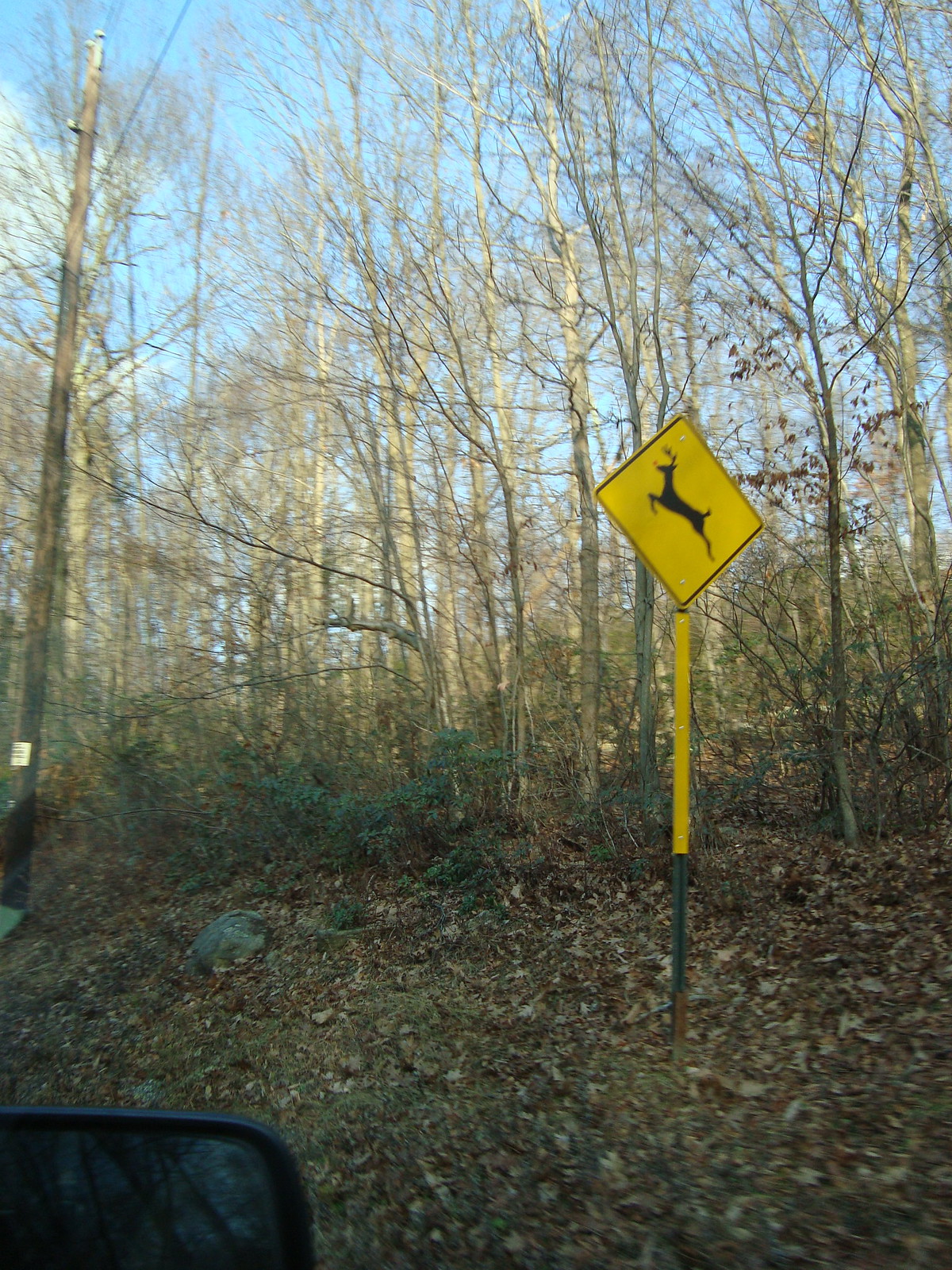The image depicts an outdoor wooded area taken from the passenger side of a car, with part of a black-framed side mirror visible in the bottom left-hand corner. The photo is slightly blurry and out of focus, likely captured with an older camera or phone. Central to the image is a patch of light green-yellow grass dotted with brown, dead leaves. Rising from this area is a green metal post topped with a yellow diamond-shaped sign featuring a black silhouette of a leaping deer, indicating a deer crossing. The background showcases a line of bare, leafless trees through which patches of a bright blue sky with wisps of white clouds are visible. A few green smaller plants are seen at the base of the sign, adding to the scene’s detail.